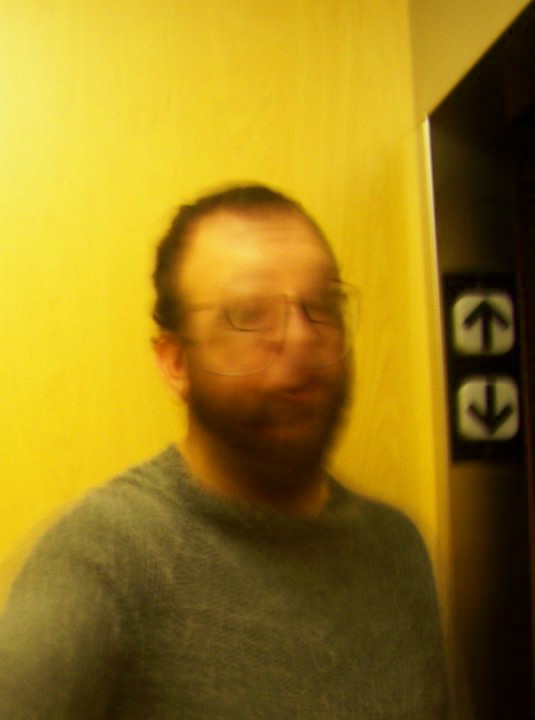The image depicts a blurry, low-quality close-up of a bearded white man in his 30s with short, dark brown hair and wire-rimmed glasses. He appears to be wearing a gray or possibly green shirt, though it is difficult to distinguish the sleeve length due to the blur. The man's face is obscured by motion blur, making his facial features unrecognizable. He occupies around half of the frame and is situated in front of an elevator, identifiable by the black up and down arrows next to the door. The background is a yellowish hue, contributing to the photo’s overall indistinct and poorly-lit appearance.